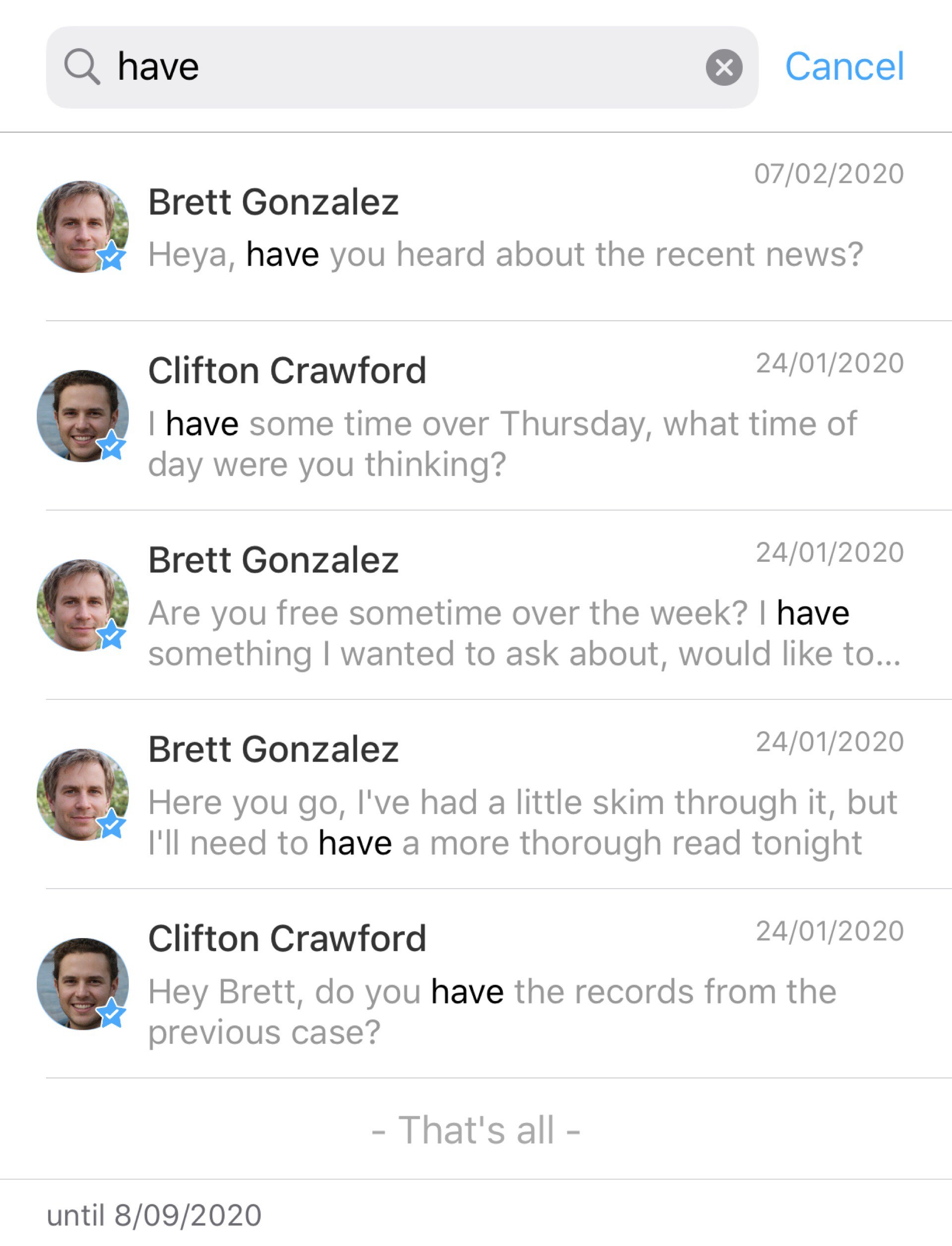This image is a screenshot from a website featuring a prominently displayed search bar at the top. The search bar is in a light gray tone and includes a magnifying glass icon and the text "have" (H-A-V-E) inside. To the right of the search bar, there is a dark gray circle with an X in the center, accompanied by the word "Cancel" in blue text with a capital C.

Below the search bar, there are five messages displayed. The first message is from Brent Gonzales, stating, "Hey, have you heard about the recent news?" Clifton Crawford responds, "I have some time over Thursday. What time of day were you thinking?" Brent Gonzales then asks, "Are you free sometime over the weekend? I have something I wanted to ask about," where the word "have" is in dark text, followed by a truncated phrase indicated by "dot, dot, dot." 

Brent Gonzales continues, "Here you go, I have had a little skim through it, but I'll need to have a more thorough reasoning," with the word "have" in dark text. Finally, Clifton Crawford replies, "Hey Brent, do you have the records from the previous case?" where again the word "have" appears in dark text. The descriptive text concludes with "that's all."